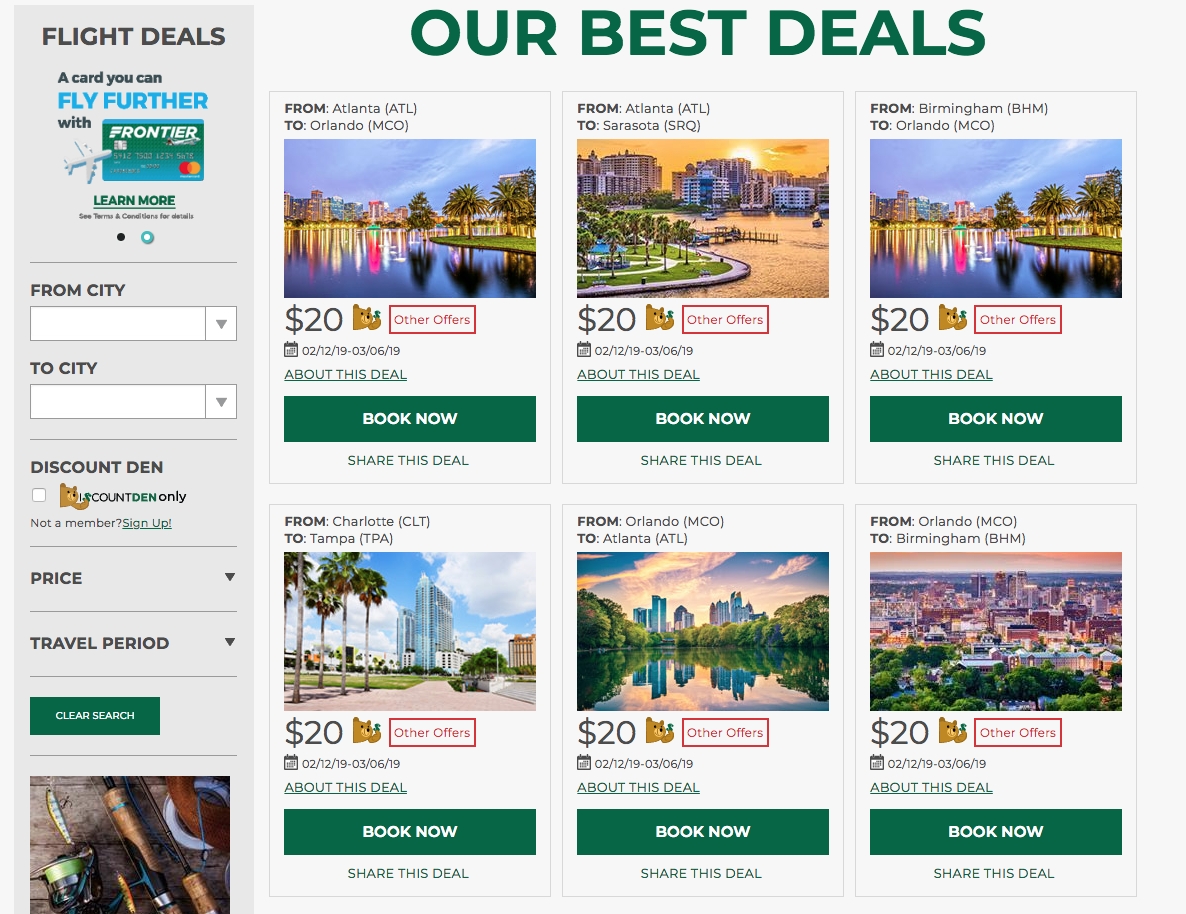**Caption:**

The image showcases a "Flight Deals" page brimming with enticing offers. At the very top, on a light gray or pale green background, the headline “OUR BEST DEALS” is prominently displayed in green capital letters. Just below, on the left side, the main section titles emerge in black text, segmented by different hues:

- **Header:** "FLIGHT DEALS" in black text.
- **Subheader:** "Fly further with" in a mix of black and blue text, featuring an image of a Frontier credit card. The credit card has a green-to-blue gradient, Frontier's logo, a MasterCard logo on the right, and a white airplane icon on the left.
- A hyperlink "Learn more" in underlined green text.
- A note in black text, "See terms & conditions for details," followed by a black dot and a teal dot highlighting the selected status.

Beneath this, the form interface includes:

- "From City" with a drop-down box.
- "To City" with another drop-down box.
- "DISCOUNT DEN" in all caps black text with a checkbox and bear icon beside it, followed by "DEN ONLY."
- A prompt, "Not a member?" with a green underlined "Sign Up!" link.
- Drop-downs for "Price" and "Travel Period," each with a black triangular arrow.
- A green rectangular "CLEAR SEARCH" button.

Below the form, a horizontally oriented image of fishing rods appears, creating a thematic backdrop for travel adventures.

The deals section features six travel offers displayed in two rows of three cards each:

1. **From Atlanta (ATL) to Orlando (MCO):**
   - Image: Tropical trees and hotels reflecting in water.
   - Price: $20 with a bear icon.
   - Dates: 02/12/19 to 03/06/19.
   - Links: “About this deal” (green, underlined), and a green “BOOK NOW” button with white text, followed by "Share this deal" in green text.

2. **From Atlanta (ATL) to Sarasota (SRQ):**
   - Image: Sunset behind hotels, water, and tropical trees with grass in front.
   - Same price and dates as above.
   - Identical link and button details.

3. **From Birmingham (BHM) to Orlando (MCO):**
   - Price and dates mirrored as above.
   
4. **From Charlotte (CLT) to Tampa (TPA):**
   - Image: Palm trees, tall hotels, blue skies, and fluffy clouds.
   - Same price and dates as previous offers.

5. **From Orlando (MCO) to Atlanta (ATL):**
   - Image: Buildings with trees reflected in water.
   - Same price and booking options.

6. **From Orlando (MCO) to Birmingham (BHM):**
   - Image: Skyline with trees closer to the camera.
   - Consistent price and dates, with standard booking details.

Each offer is meticulously detailed, presenting a visual treat and easy-to-navigate booking options for potential travelers.